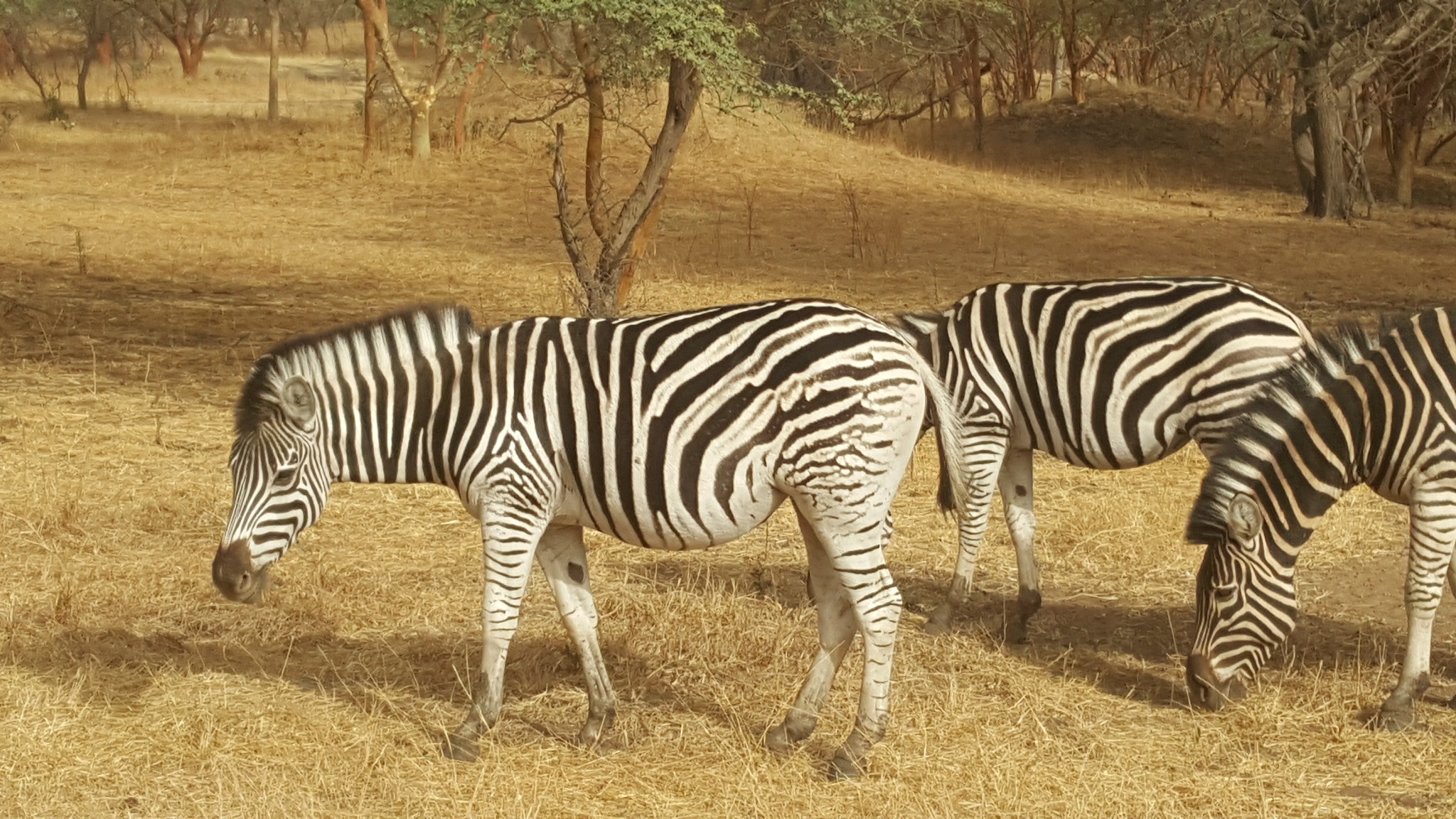The image captures an outdoor scene bathed in bright sunlight featuring three zebras in a dry, grassy area with sparse trees in the background. The central focus is a fully visible zebra slightly left of center, standing in profile with its head pointed down toward the left corner of the image. The grass beneath them is a tan, prairie-like terrain, dry and mostly brown. Behind this central zebra, another zebra's body is partly visible, although its head is obscured by the zebra in front. The third zebra appears on the right edge of the photo, with its head also down towards the grass and only its head and one front leg visible. The scattered trees in the background have a few green leaves, indicating a sparse, arid environment. The sunlight from the right casts slight shadows of the zebras toward the front. Notably, the third zebra has thicker and darker stripes compared to the other two. The overall composition, with all zebras facing left and the detailed interactions between them, vividly captures a moment in their natural habitat.